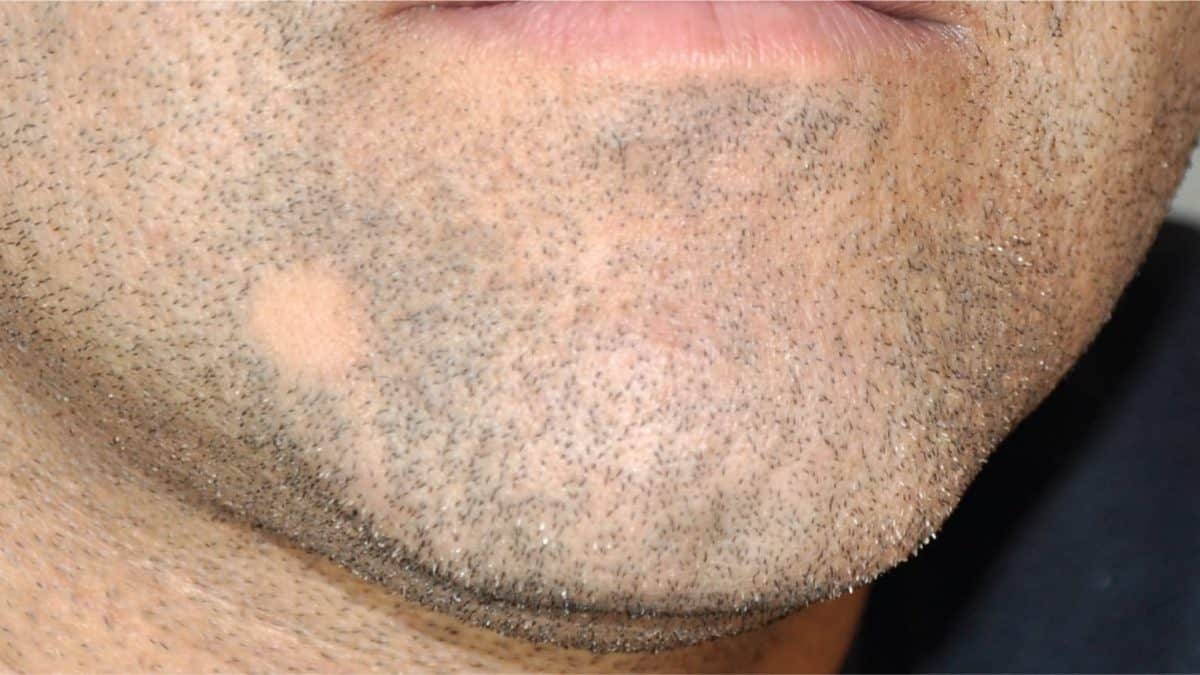This image is a close-up, rectangular photograph focused on the chin of a white, unshaven man. His lower lip is visible at the top of the image, while the beginnings of his neck can be seen at the bottom, although most of his facial features are out of frame. The man's chin is covered in stubble, suggesting he hasn't shaved for a couple of days. Notably, there is a small spot on the left side of his chin, about half an inch wide, where no hair grows, possibly due to a scar. The background shows a hint of blue, likely a wall, but this is mostly obscured by the man's face, which fills almost the entire frame. The overall setting and positioning suggest that the image was likely taken casually, possibly at home, to examine the stubble up close. The predominant colors in the image are various shades of pink, black, tan, and blue-gray. The man is unsmiling, adding to the photo's introspective feel.